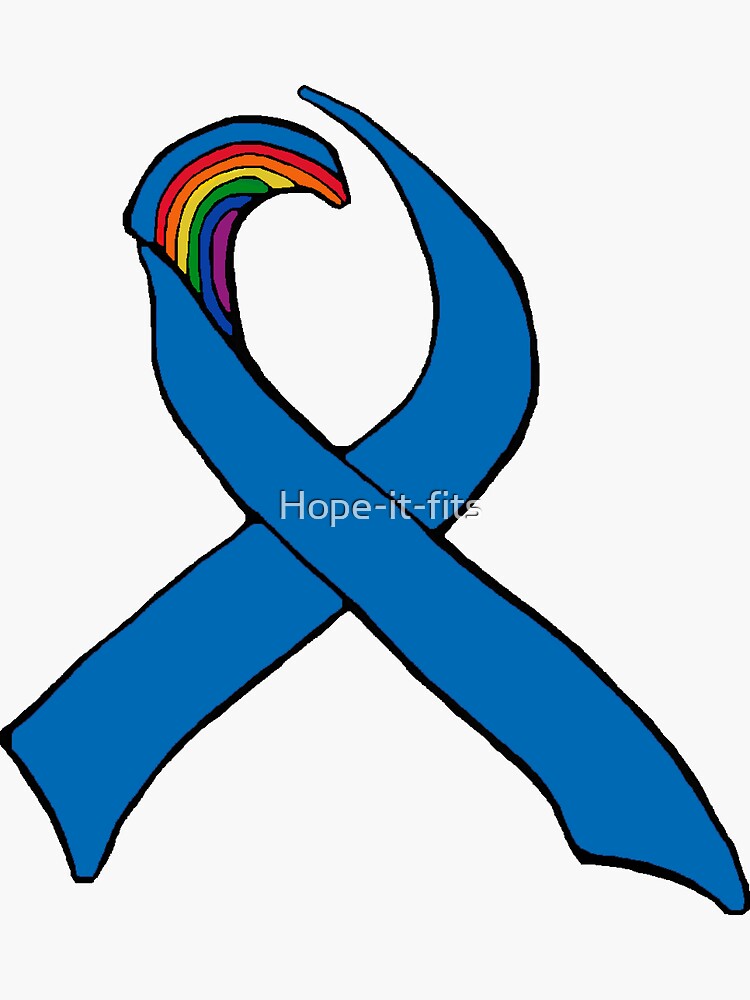The image is an illustration of a dark blue ribbon, similar to those used for symbolic causes such as breast cancer or LGBTQ awareness. The ribbon, outlined in black, is positioned against a light gray, almost white, background with no other elements in the frame. At the top of the ribbon, the inner edge features a vibrant rainbow design with stripes in red, orange, yellow, green, blue, and purple. The ribbon forms a loop at the top with the two ends hanging down and crossing at the bottom. Centrally placed over the ribbon, in a light gray translucent font, the text reads "hope-it-fits," hinting at the idea of fitting into or supporting a cause. No people, animals, or natural settings are present, focusing attention solely on the cause symbolized by the ribbon and the hopeful statement in the foreground.